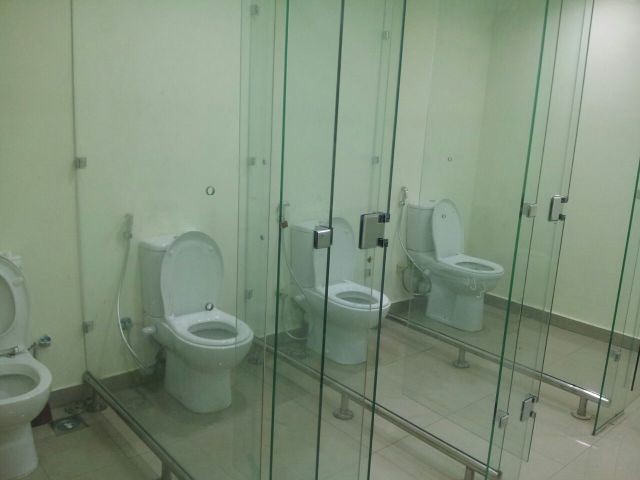This image depicts a modern, somewhat unconventional bathroom with four white porcelain tank-type toilets arranged in a row, slightly diagonally from the lower left to the center right. Each toilet is enclosed within individual stalls made of completely see-through glass panels, which are supported by stainless steel metal bars at the bottom. The stalls feature metal latches on their doors, which are all currently open. A hose-like tube is visible to the top left of each toilet, connecting to the wall. While the seats on the three toilets to the right are down, the one on the far left has its seat up. The background consists of solid white walls, and the floor is covered with large, reflective, light brown ceramic tiles. The overall setting exhibits a greenish cast from the fluorescent lighting present in the room. There are also small metallic contraptions noted on the floor near the partially cut-off toilet on the left-most side of the image.